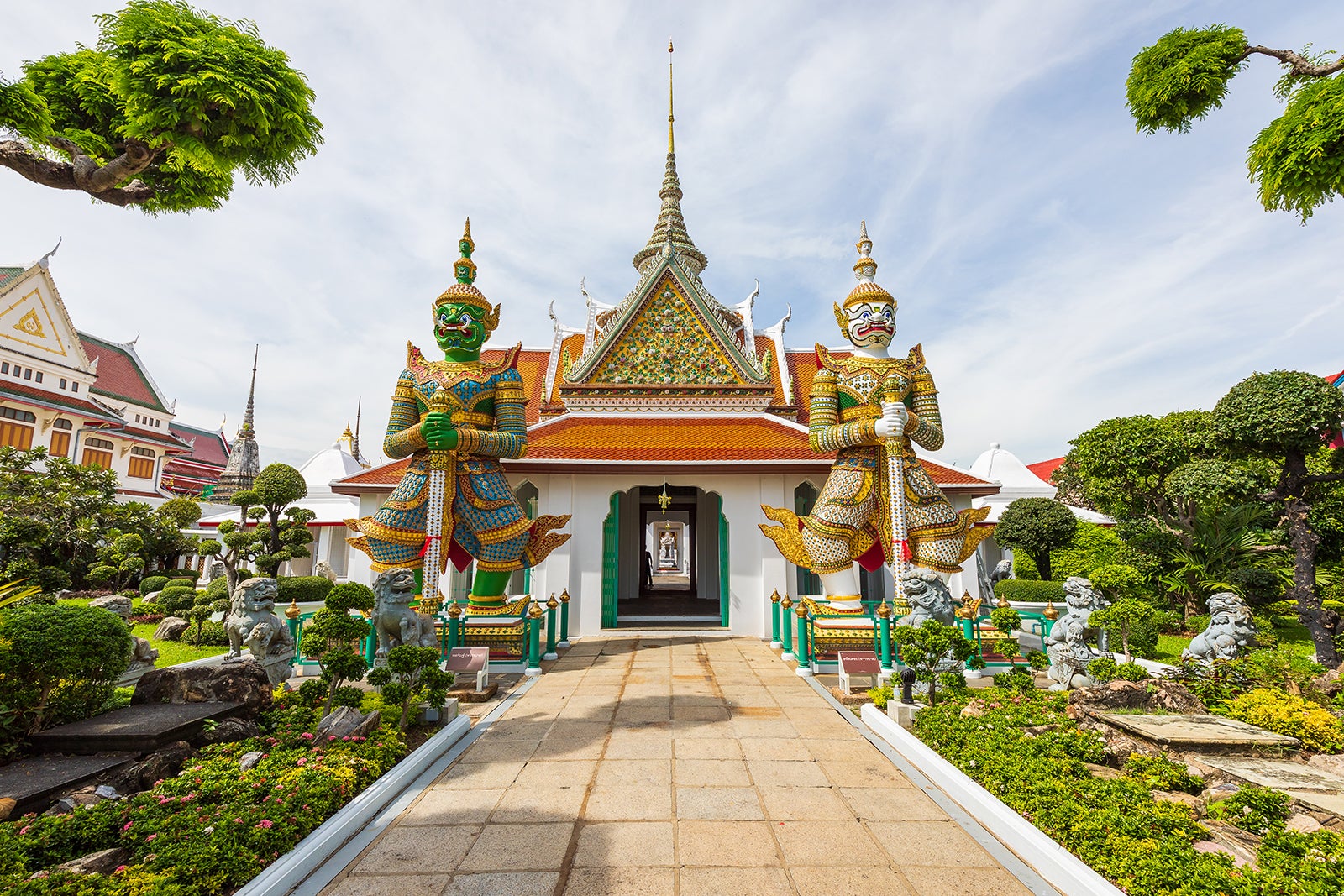This detailed image depicts a picturesque Southeast Asian temple surrounded by lush, manicured gardens featuring miniature trees reminiscent of bonsai. The temple's architecture is striking, characterized by a slanted roof adorned in alternating hues of red, orange, and white, with a central, triangular, green and yellow facade that culminates in a golden spire. An arching open doorway invites visitors into the building.

Flanking the temple's entrance are two imposing, life-sized statues that stand guard. The statue on the left has a green body and a demon-like face with sharp teeth, while the statue on the right is similarly designed, but with a white body. Both statues are dressed in elaborate, ornate armor, with golden accents and a sword plunged into the ground. Additionally, there are stone lions and gated enclosures surrounding the bases of these statues to prevent any interference.

The vibrant, well-maintained gardens are rich with various green plants and shrubbery, enhancing the tranquility of the scene. A brown pathway leads directly to the temple, guiding the eye through this serene and spiritual setting. In the background, another colorful building displays purple roofs, orange doors, and gold trimmings, adding to the vibrant and exotic ambiance of the locale. The overall impression is one of a sacred, possibly religious site, distinguished by its intricate design and serene surroundings.